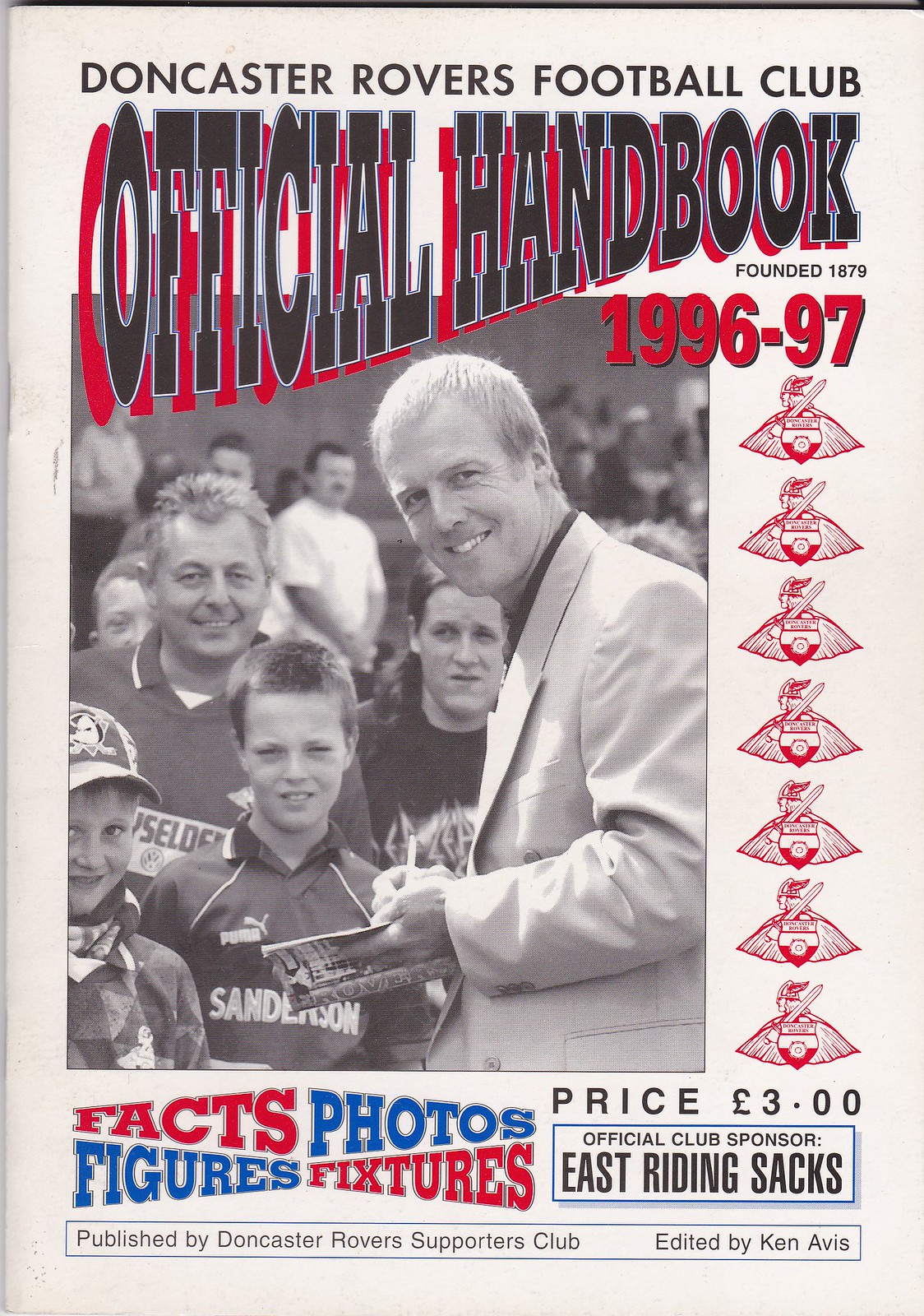The image depicts the cover of the Doncaster Rovers Football Club Official Handbook for the 1996-1997 season. The top of the pamphlet prominently displays the club's name along with its founding year, 1879, in bold text with red shadowing. Below this, a repetitive pattern of an outlined shield emblem, featuring a sword and a caped figure, runs vertically down the page until the pricing information at the bottom, marked £3. To the left of the emblem pattern, a black-and-white photograph captures a suited man, possibly a club official or player, smiling and signing the handbook for a group of enthusiastic children in what appears to be a stadium setting. Below this photo, the text reads "Facts, Photos, Figures, Fixtures." It also lists the official club sponsor as East Riding Snacks and states that the handbook is published by the Doncaster Rovers Supporters Club and edited by Ken Avis.